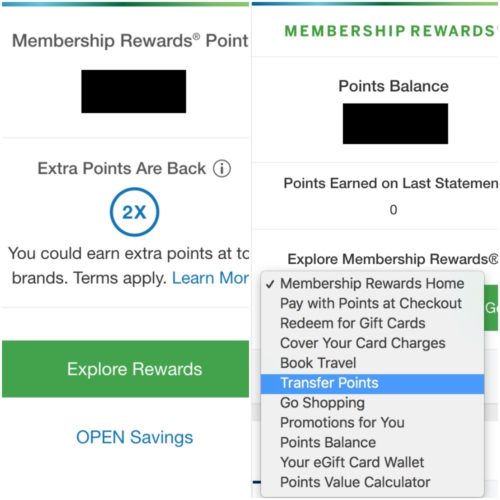The image depicts a digital screenshot or page showcasing a promotion for a rewards program. At the top, the text "Membership Rewards" is prominently displayed, followed by a bold, black bar with the announcement: "Extra Points are Back". Directly beneath, an icon resembling a coin is visible, marked with "2x", indicating that points can be earned at double the normal rate. 

The following line is partially obscured but suggests that you can earn extra points at specific brands, along with a note that terms apply. Options to learn more and explore rewards are provided.

Further down, details are listed including: "Open Savings", "Membership Rewards Point Balance", "Points Earned on Last Statement", and an invitation to "Explore Membership Rewards". The navigation options presented include "Membership Rewards Home", "Pay with Points at Checkout", "Redeem for Gift Cards", "Cover Your Card Charges", "Book Travel", "Transfer Points", "Go Shopping", "Promotions for You", "Points Balance", "Your e-Gift Card Wallet", and "Points Value Calculator".